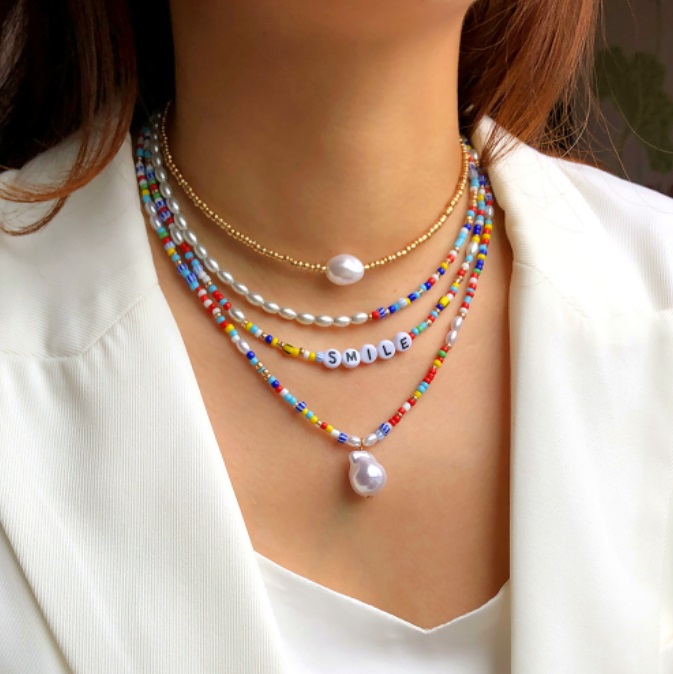This detailed color photograph, presented in a large square format, captures a close-up focus on a woman's neck and chest. The image starts from the top of her neck, where she wears a choker-style, fine gold chain adorned with a single elliptical-shaped white pearl at its center. Her neckline showcases layers of multicolored beaded necklaces, three in total. The second chain features white beads with black letters spelling "SMILE," each letter on an individual bead. The third and longest necklace, composed of small multicolored beads, culminates in a distinctive drop-shaped pearl. She is dressed in a sharp white blazer over a low-cut white blouse, highlighting her light brown, tan skin. Her straight, shoulder-length reddish-brown hair can be seen subtly framing the top left and right corners of the image. The background is a dark color, ensuring the necklaces and her attire remain the focal point of this representation of Photographic Realism and Product Photography.